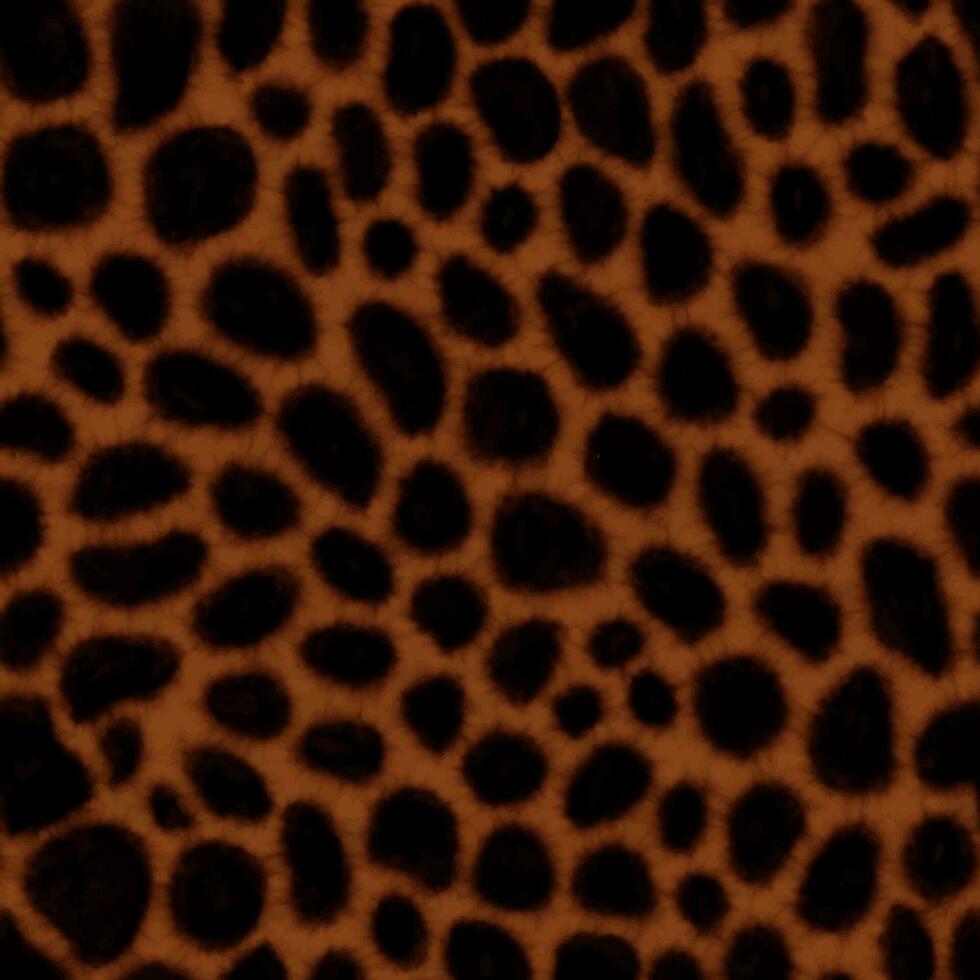The image features an intricate pattern that could be either a photograph or an AI-generated picture. Displaying a design reminiscent of a cheetah or leopard pattern, it consists of numerous black, fuzzy dots or ovals densely packed together on a dark orange or brownish background. These dots look like they could be cells or honeycombs due to their fuzzy edges and spiky details, which give the illusion of texture similar to fur. The background has a hazy, diffuse orange tone that enhances the naturalistic appearance of the pattern. Despite the detailed observation, the exact nature of the image remains ambiguous, with no text, people, or additional context provided.